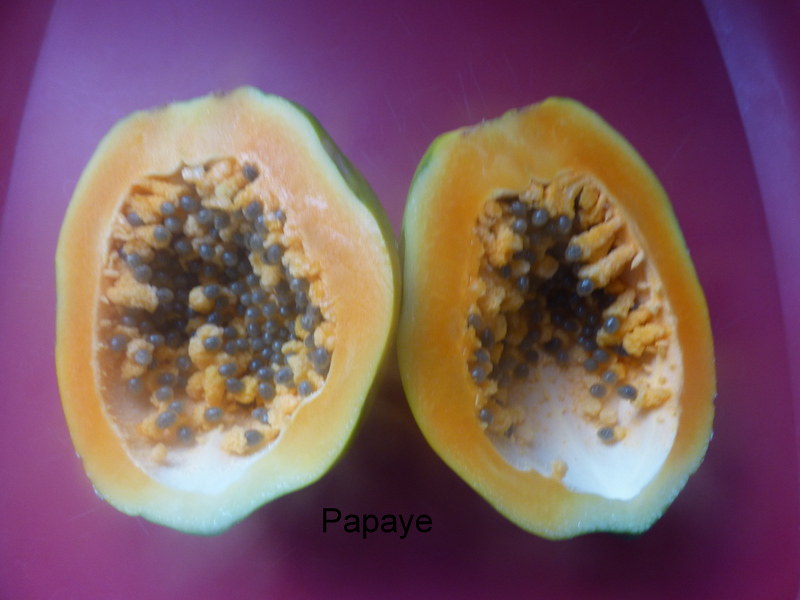This detailed image showcases a halved papaya prominently placed on a purple cutting board. The two halves of the papaya are positioned side by side, revealing their vibrant interiors. The flesh of the papaya is a rich orange color, contrasted by its grainy texture and uniquely colored seeds. Interestingly, the seeds appear to be a mix of orange and dark purple. Overlaying the image, in black text, is the misspelled word "papaye" (P-A-P-A-Y-E), located centrally at the bottom of the photo. Various color elements such as green, burgundy, orange, yellow, and black subtly pepper the background and the fruit itself, adding depth to the visual composition.